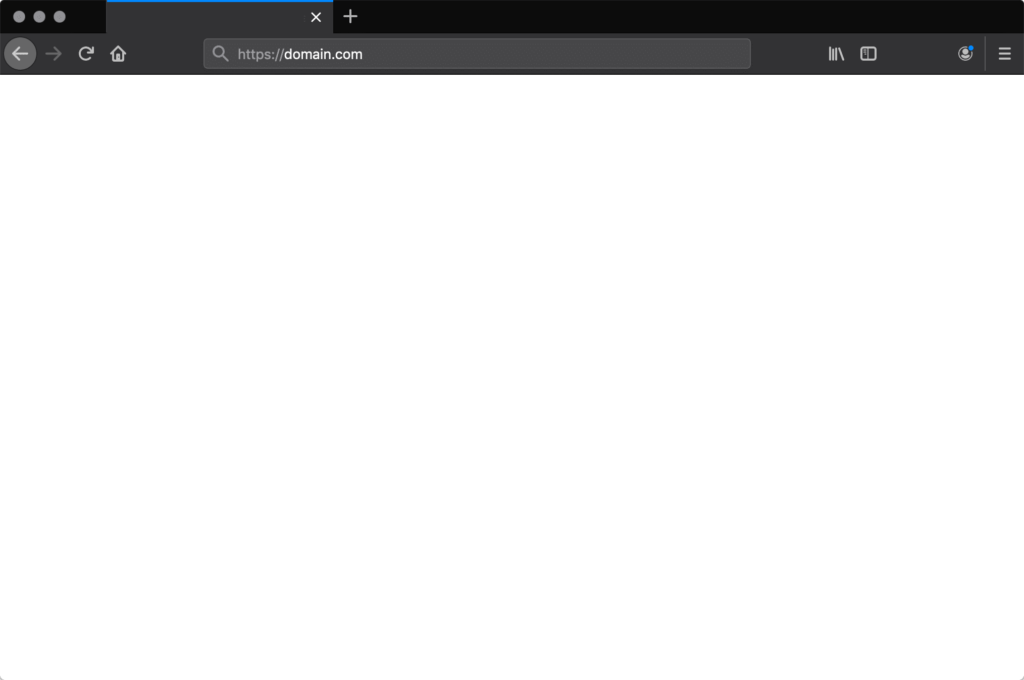The image depicts a web browser interface in a mostly black and white color scheme, with the exception of a few blue accents. At the top, there is a navigation bar featuring three circular buttons on the left, commonly associated with window control (close, minimize, maximize). The active tab has a blue horizontal highlight, indicating its selection, but bears no text. To the right of the tabs is a person icon marked with a small blue dot.

Below the tab bar is the main toolbar, which is slightly lighter in shade compared to the rest of the interface. This toolbar contains several browser icons: a back arrow encircled, a forward arrow, a reload button, a home button, and a field displaying the URL "https://domain.com". Additionally, there are icons for bookmarks (depicted as three bookshelves), a square (possibly for apps or extensions), another person icon with a blue dot, and a hamburger menu (three horizontal lines).

The majority of the browser window is a blank, white page with no content, reinforcing the impression that this is an example or template of a browser setup. The choice of the blank page suggests it may have been intended to serve as a basic illustration of a browser interface, but inclusion of a test page might enhance its utility for demonstration purposes.